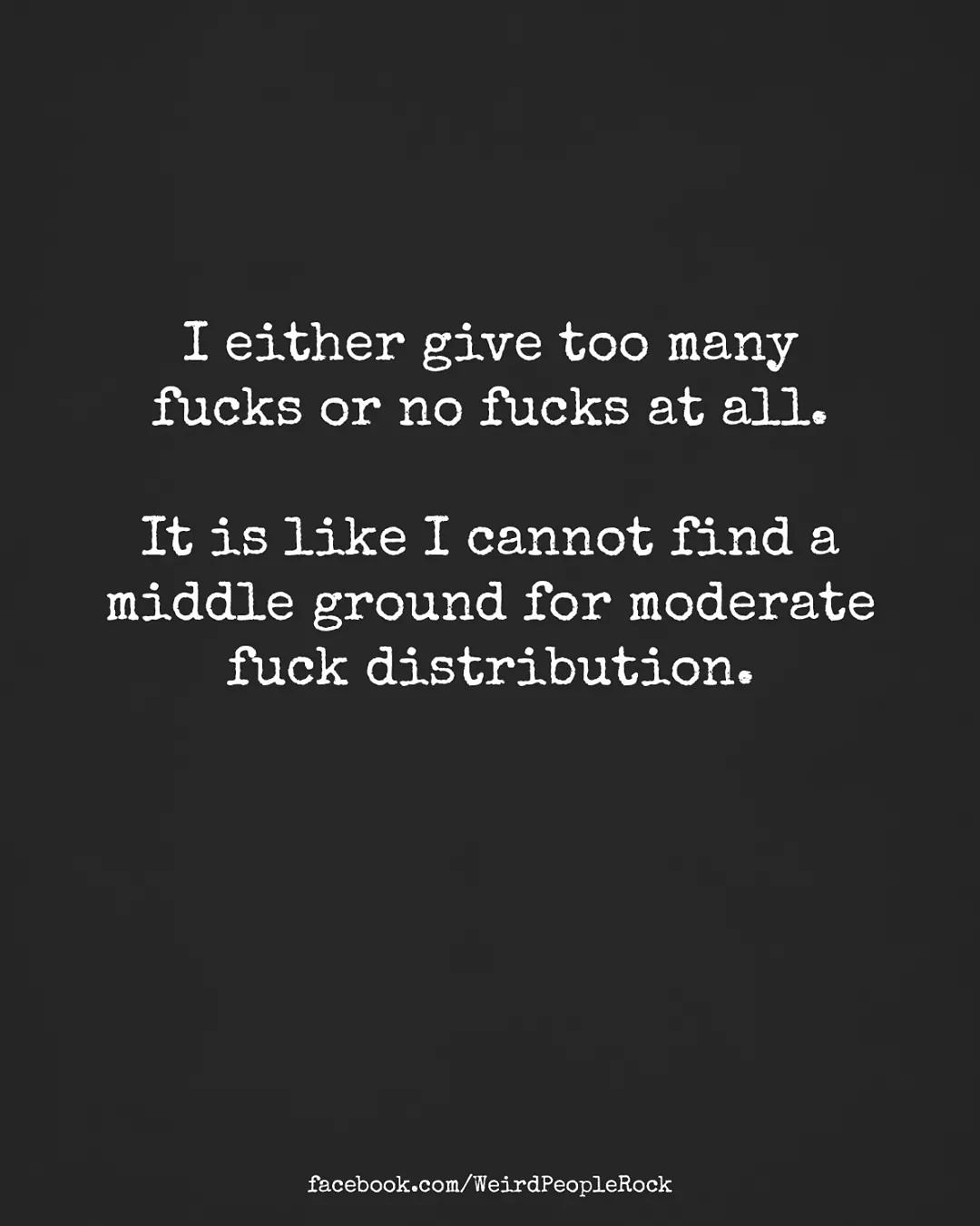The image features a stark, minimalistic design with a solid black background and white text in a basic, typewriter-like font. The text reads, "I either give too many fucks or no fucks at all. It is like I cannot find a middle ground for moderate fuck distribution." At the bottom of the image, it says "facebook.com/weirdpeoplerock." This simple yet impactful presentation likely didn't require much time to create but conveys a strong sentiment about the inability to find balance in caring.